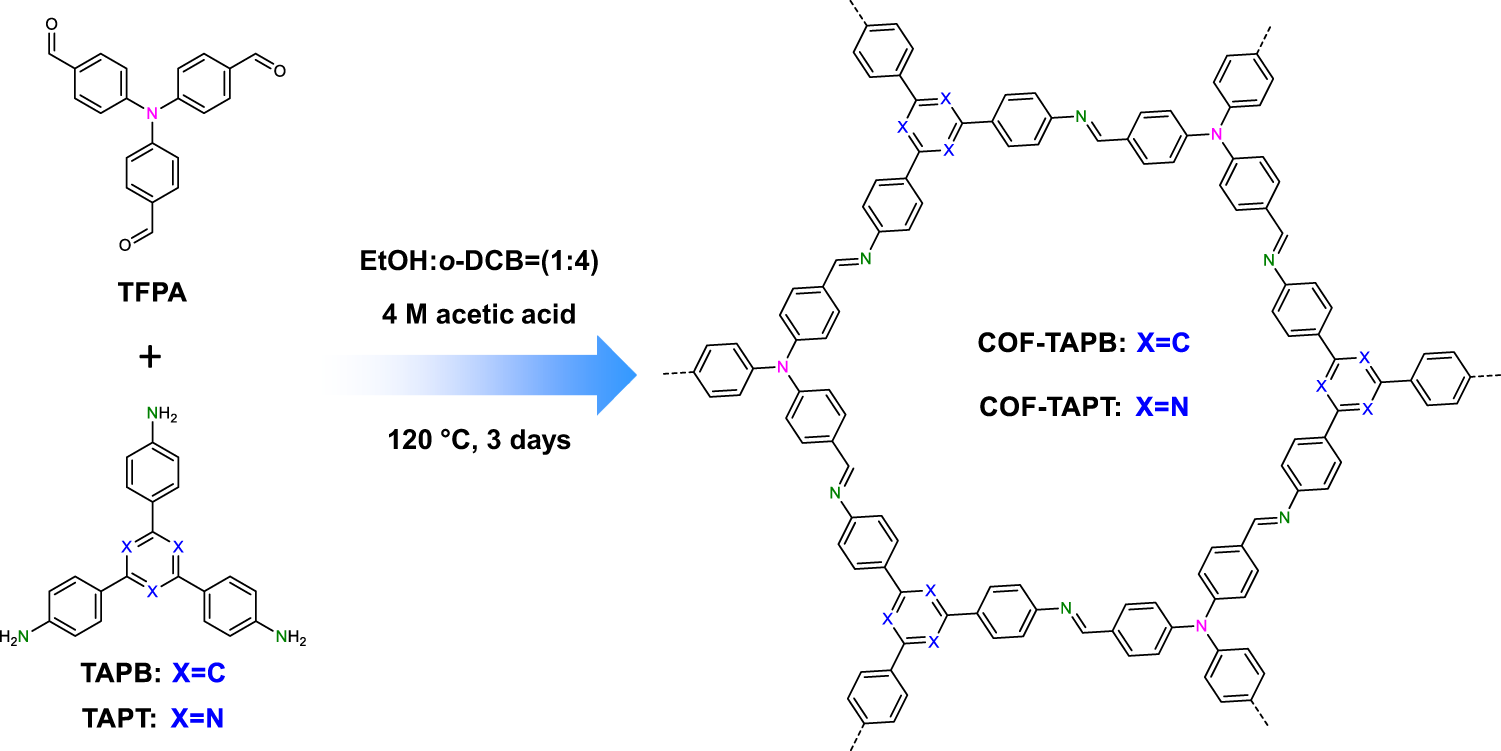The image portrays a scientific diagram featuring molecular structures composed of interconnected black-and-white hexagons. Central to the image are two smaller clusters of polygons, positioned vertically on the left, with text between them reading "TFPA" above, and "TAPB X = C" and "TAPT X = N" below. Adjacent to these, there are chemical reaction conditions: "ETOH, DCB = 1 to 4, 4M acetic acid, 120°C, 3 days." A prominent blue arrow points to the right where the most complex molecular structure is displayed, forming a large polygon from numerous smaller ones. The colors visible in the image are predominantly blue, light blue, black, and white, suggesting a digitally rendered illustration.